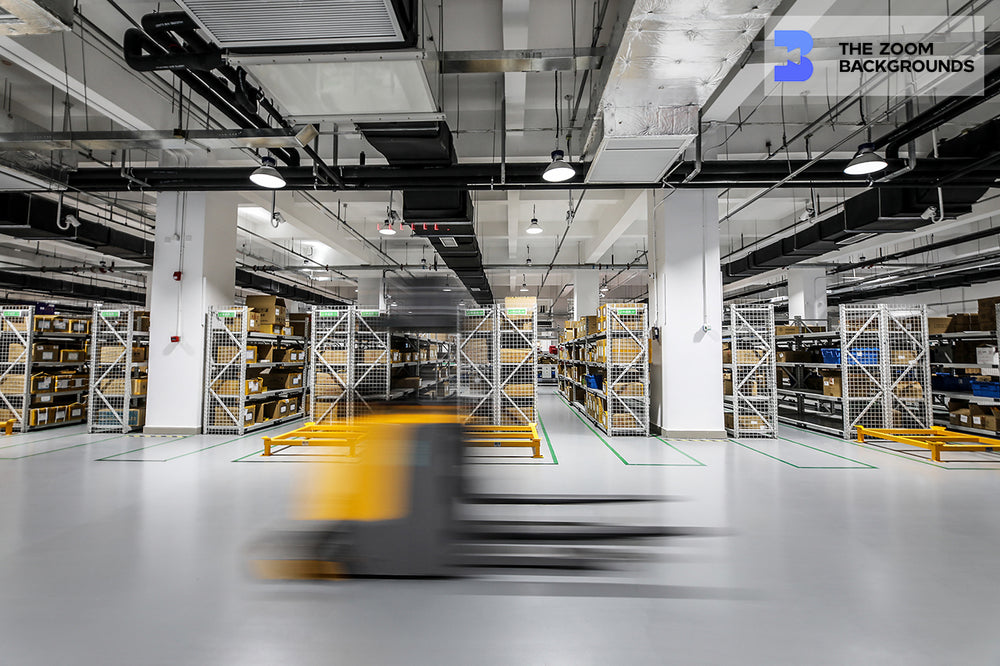The image depicts an extremely clean, large warehouse with a slick, light gray floor. Rows of metal shelves filled with labeled boxes are neatly arranged between big white pillars that support the ceiling. Overhead, silver beams and horizontal black bars intersect the ceiling, which is adorned with pendant lights and a combination of black and silver ductwork, creating a well-lit and organized environment. The ceiling itself is prominently silver, contributing to the overall industrial aesthetic. Near the bottom of the image, a fast-moving machine in yellow and gray—likely an automated forklift—appears blurred with motion lines trailing behind it. In the top right corner, a transparent white rectangular box reads "The Zoom Backgrounds" in black text, accompanied by a logo resembling a bee with a camera on the left side.